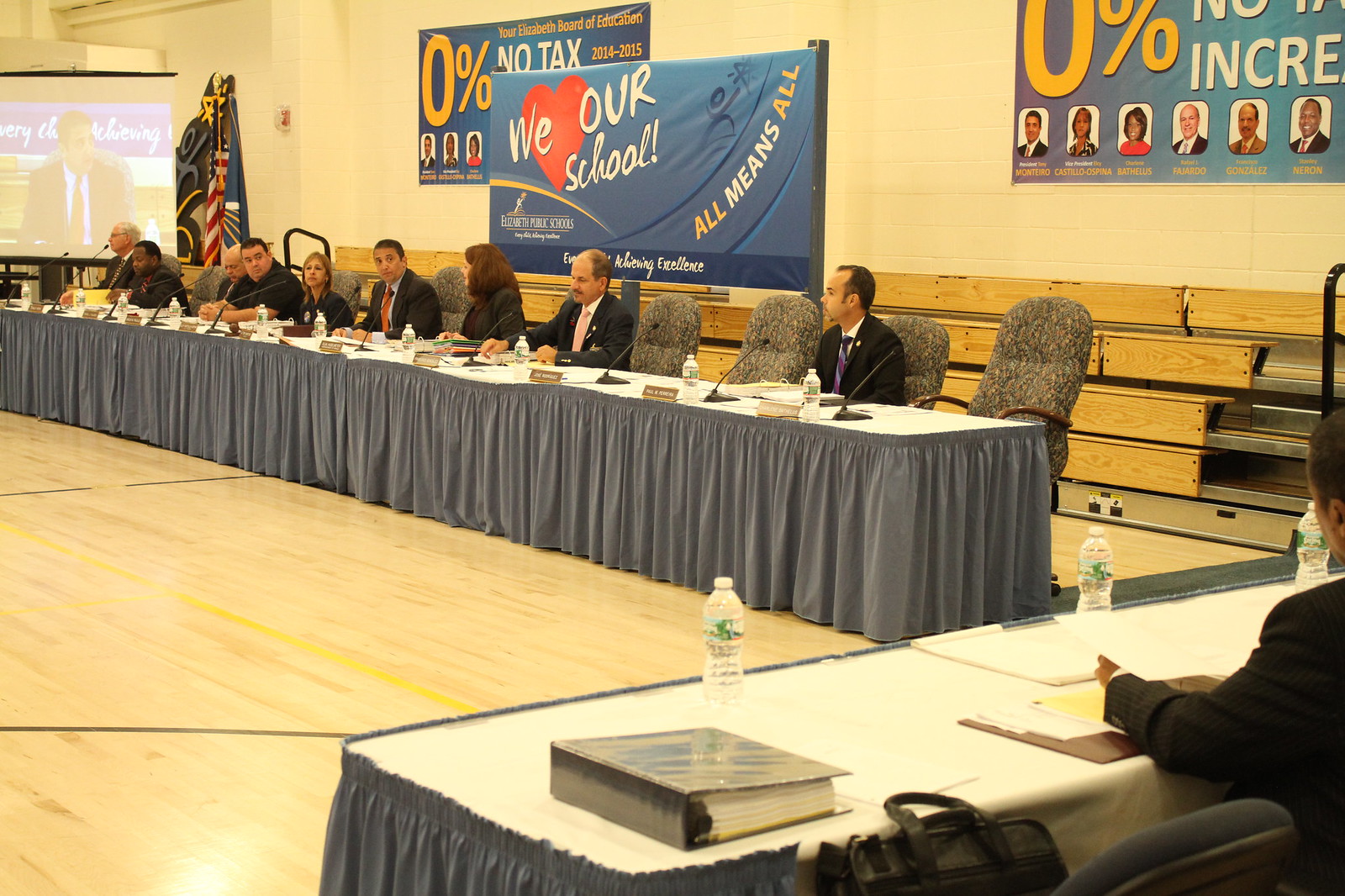This is a color photograph taken inside a school gymnasium, easily identifiable by the wooden bleachers that are pushed against the wall in the background and the hardwood basketball court floor. Two long tables dominate the scene, each covered with a white tabletop and draped with long gray skirts. Arranged around these tables are executive office chairs, many occupied by individuals in business attire, primarily men in dark suits. Each seating position is equipped with a microphone, a corresponding nameplate, a large notebook, and a small plastic water bottle. In front of them, a banner hangs that reads, "We Love Our School. All means all." In the far left upper corner, a projector screen displays an image of a man in a suit, seemingly addressing the attendees. Additionally, in the corner of the gymnasium, an American flag is visible. Another smaller banquet table appears in the foreground, manned by individuals who do not have microphones or nameplates, possibly secretaries documenting the meeting. The overall setup and formal atmosphere suggest that this is a school board meeting being held in the gymnasium.